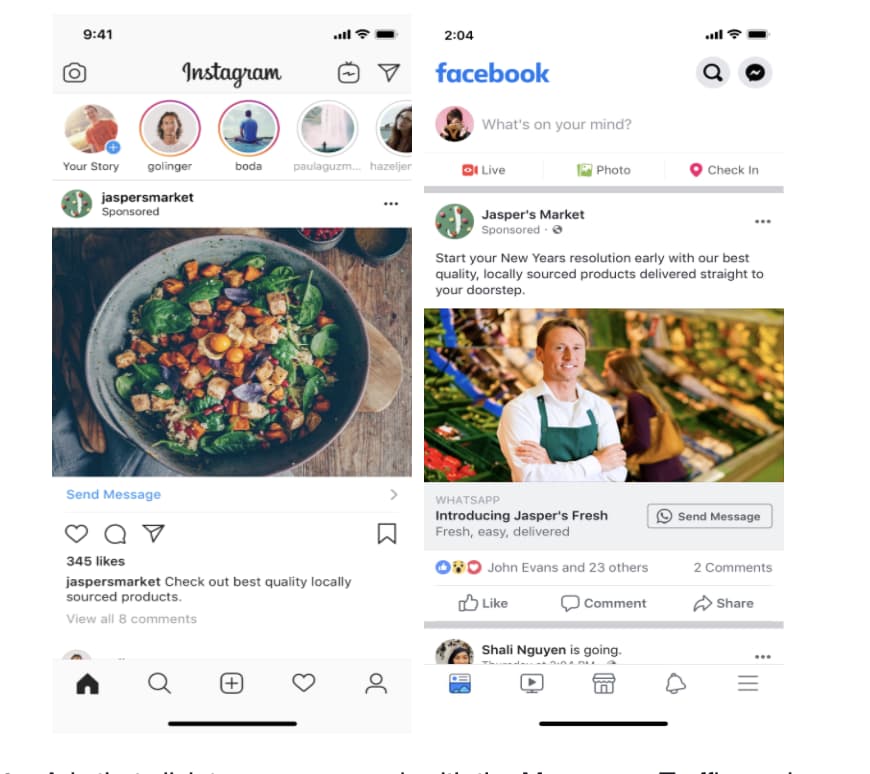The image contains two sets of screenshots: one from the Instagram app and one from the Facebook app.

In the Instagram screenshot, the status bar reads 9:40 with a strong cellular signal, full Wi-Fi, and a fully charged battery. The interface includes the classic camera icon and the Instagram logo along with a squiggly line icon and a send button. There are five profile circles at the top: "Your Story," "Goinger," "Boda," "Paradigm," and an empty spot. Below these, there's a sponsored post by "Jasper Market" featuring a close-up of a colorful salad plate. Interaction buttons underneath include a heart, a conversation bubble, a send/share icon, and a bookmark. The post has 305 likes and a caption by Jasper Market: "Check out best quality locally sourced products." Additionally, there are eight comments visible.

In the Facebook screenshot, at the top is the prompt "What's on your mind?" followed by options for "Live," "Photo," and "Check-in." Below these options, there’s another sponsored post by Jasper Market. The post encourages users to "start your New Year's resolution early with our best quality locally sourced products delivered straight to your doorstep." It features a picture of a white gentleman wearing a long-sleeve white shirt and a green apron. Beneath this image is the heading "Introducing Jasper's Fresh" with a "Send Message" button.